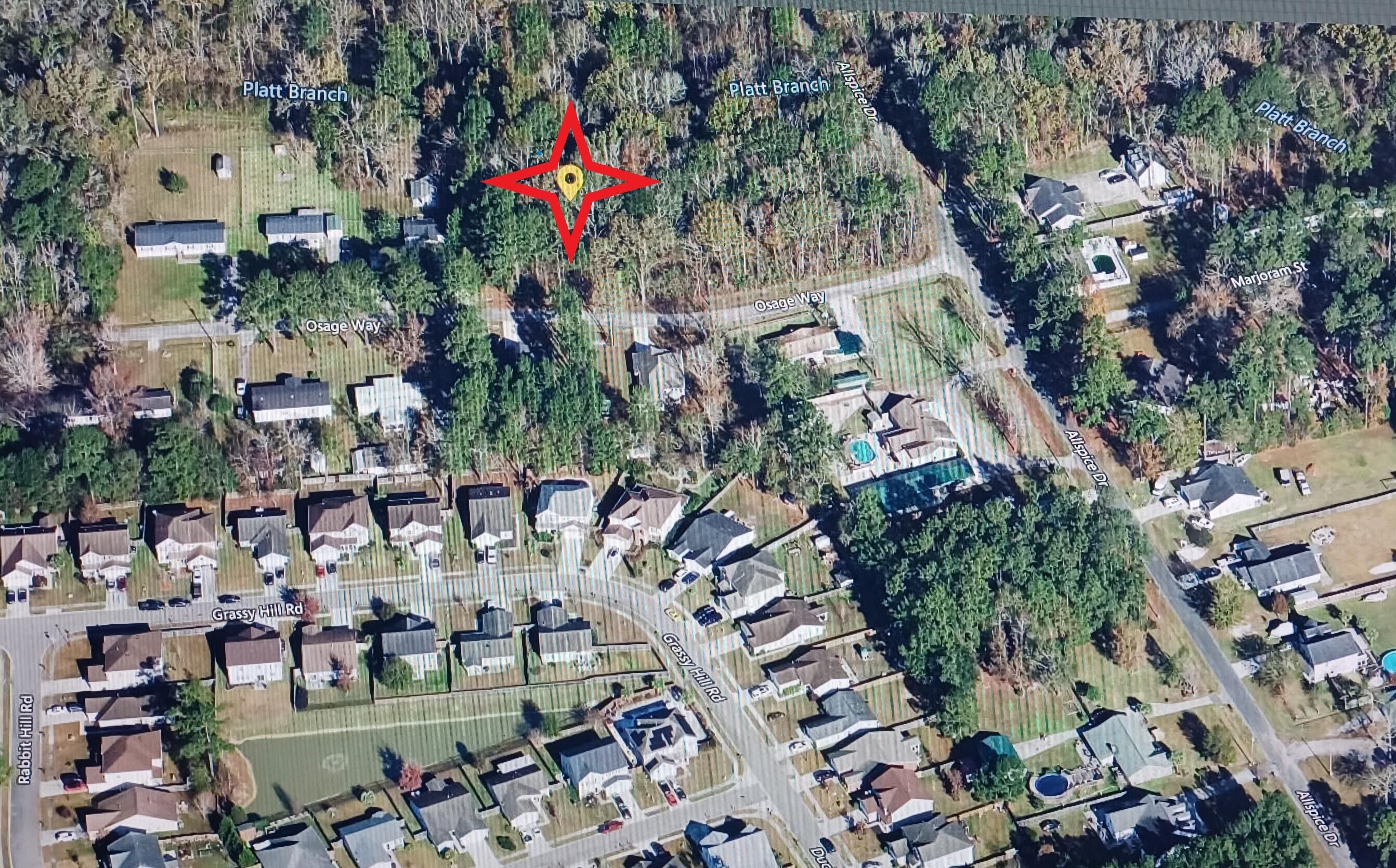This image appears to be a detailed Google Maps screenshot showcasing an aerial view of a residential neighborhood with a cul-de-sac layout and a surrounding subdivision. Prominent road names such as Platten Branch, Osagie Way, and Majeram Street are visible, aiding in navigation. The focal point is a yellow pin with a red-star outline, possibly marking a piece of land for sale amid a few empty lots. The neighborhood is characterized by a fanned pattern of identical houses, accompanied by a central triangular cluster. Various homes feature blue swimming pools in their backyards, contrasting vividly with the lush green foliage of the trees, some of which are beginning to show autumn colors. Additionally, a central lake with greenish water is a notable landmark within the community. The image captures various colors including blue, green, tan, black, gray, and pink, contributing to the vibrant depiction of this residential area.